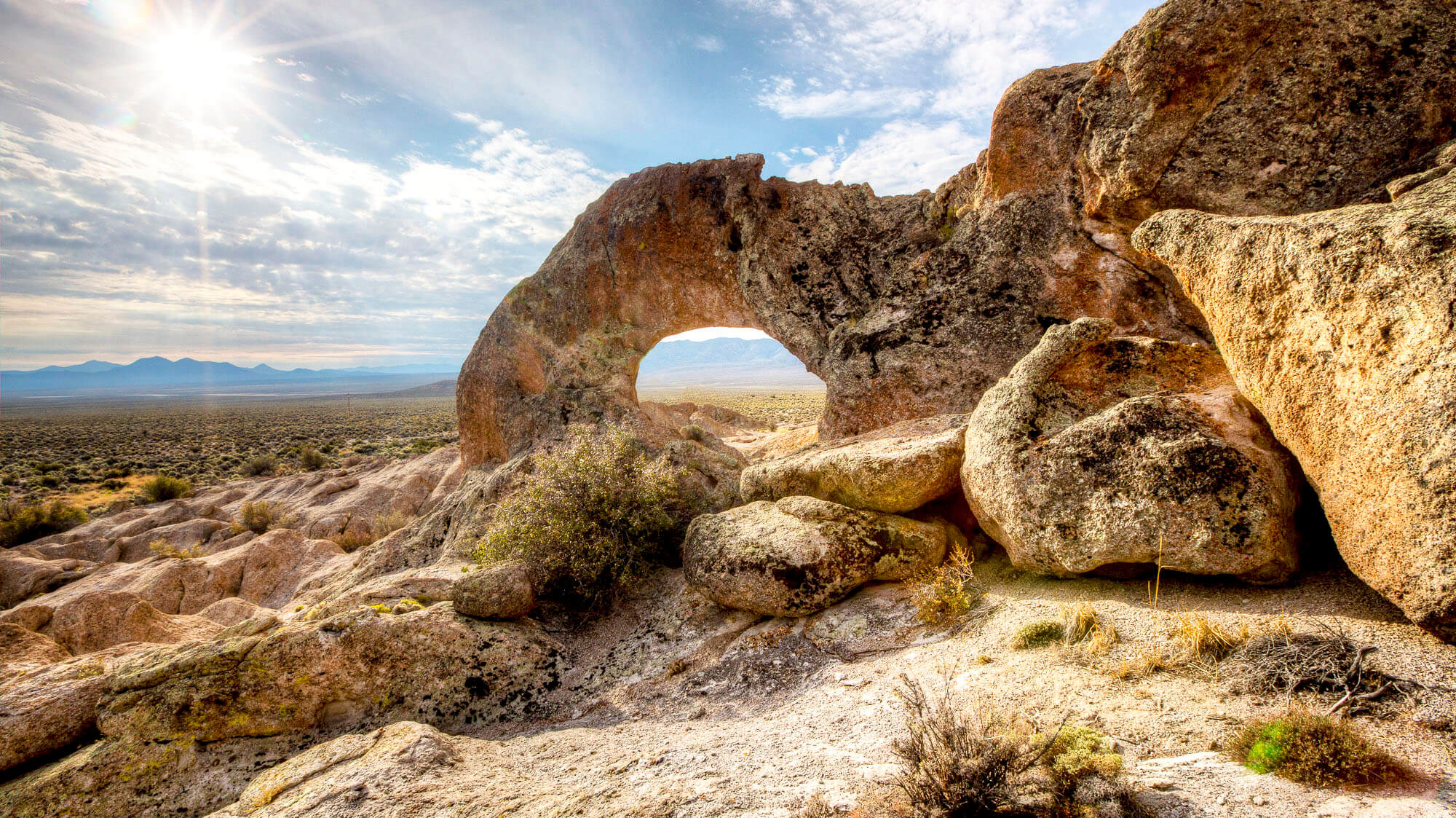The image captures a sunny day in the desert southwest, highlighting a striking and somewhat unique rock formation. In the foreground, the eye is immediately drawn to a large rock formation featuring an arch or "rock doughnut" with a hole through which distant mountains are visible. Wispy clouds float in a blue sky, through which rays of sunlight beam down, illuminating the barren, desolate landscape. Vegetation is sparse—only a few small bushes and desert plants cling to life, displaying shades of green mixed with tans, browns, and yellows. The area is dominated by rocky terrain, including both large climbable structures and smaller rocks scattered across the foreground. In the background, the expansive landscape stretches out, with the rugged mountains and a hint of greenery. This dry, remote location seems perfect for adventurous hikers, a place where one must surely stay hydrated.